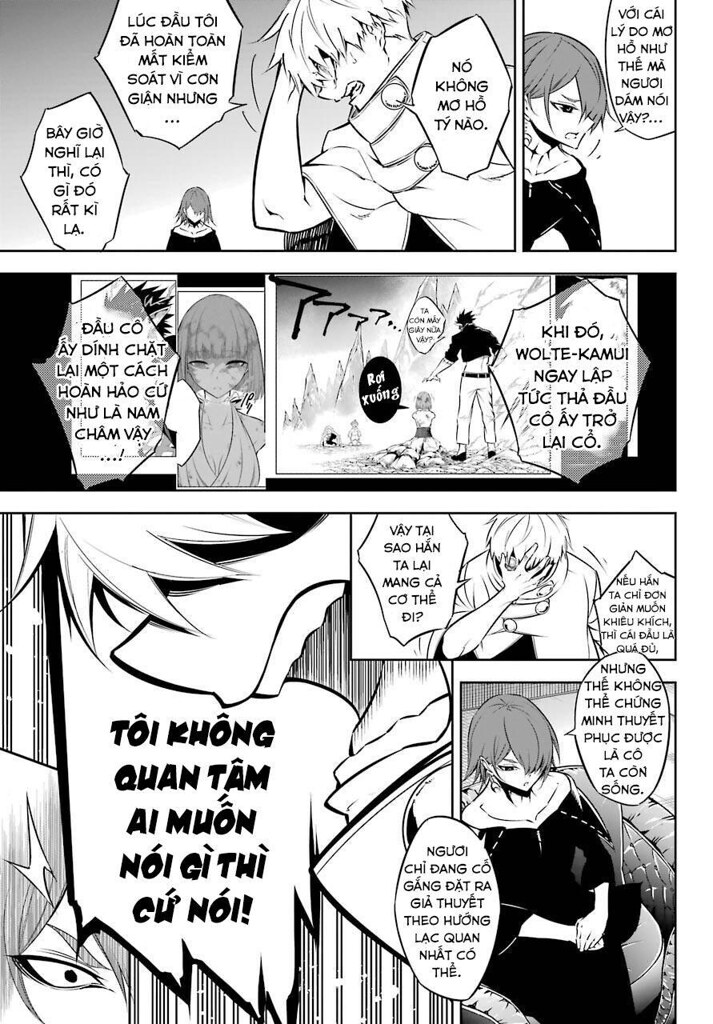This black-and-white comic strip appears to be a page from a manga and is composed of three vertically stacked panels, each depicting intense interactions between the characters. The dialogue seems to be written in a foreign language, possibly Vietnamese. 

In the first panel on the top right, a female character with dark, short hair is speaking vehemently. Opposite her in the upper left panel, a man with white hair responds, also speaking intensely. The scene then transitions to a different setting in the third panel, showing another female character with lighter hair and yet another woman with dark hair. This new pair also appears to be in their own intense dialogue. 

Returning to the earlier conversation, the tension escalates in the lower panels. The white-haired man is depicted clutching his face, showing visible distress, while the dark-haired woman responds, her intense expression suggesting she's deeply engrossed in the conversation. In the final box, the man, now shouting, says something that visibly shocks the woman. Overall, the sequence conveys a complex, tension-filled storyline involving multiple characters caught in intense exchanges.